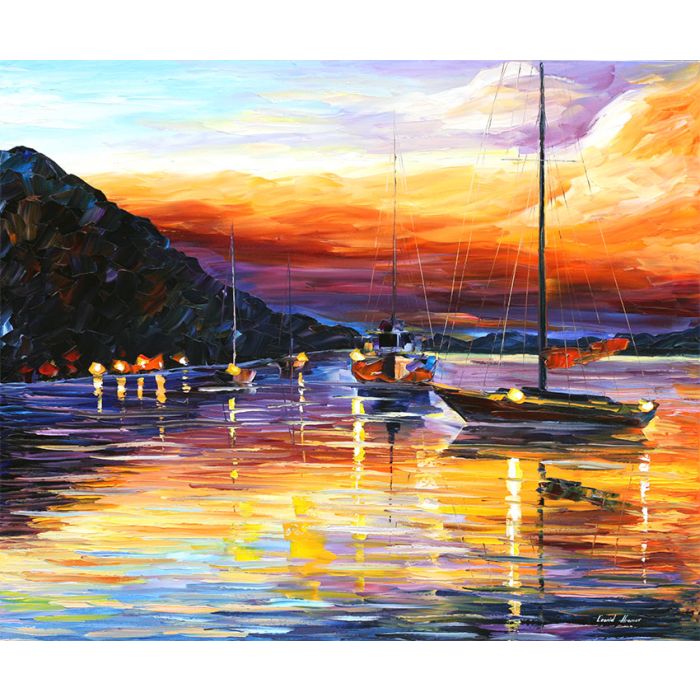This is an abstract, impressionistic painting depicting a serene boat scene. The water at the bottom is a vibrant mix of yellow, red, blue, and green created with horizontal streaks. Within this colorful expanse, several small sailboats rest with their sails down and masts pointing straight up, framed by the crisscrossing lines of their ropes. Dominating the right side of the painting, one boat's broadside faces the viewer, while the other sailboats, positioned to the left, include a larger boat in the center and two smaller ones further left, all facing the viewer's perspective.

On the left edge of the composition, a prominent rocky outcropping, resembling a slice of pizza laid on its side, features striking blue and purple highlights on an otherwise dark gray and black surface. Above, a beautifully streaked sky mirrors the water's colors, transitioning from deep purple at the base to warm orange in the middle, with the top left showing shades of blue and the top right tinged with purple. This harmonious blend of colors, reflecting a likely sunset, bathes the entire scene in an ethereal light.

In the background, low-lying rocks seemingly restrict the boats from sailing further, suggesting a calm harbor setting. Enhancing the painting's originality, a signature is visible at the bottom right corner.